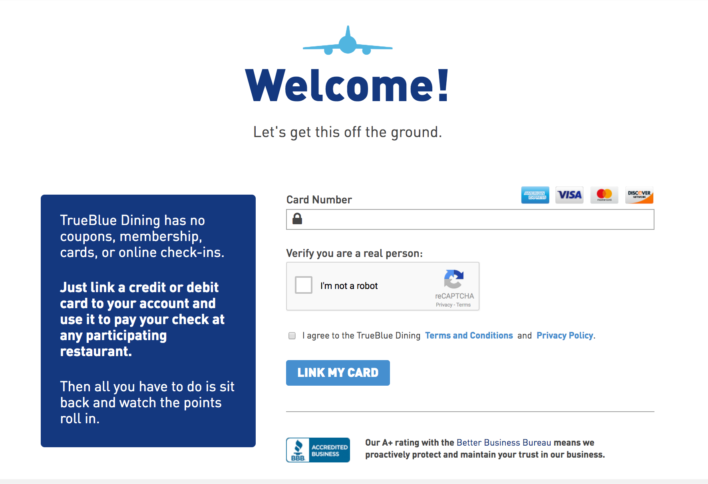The image features a webpage from the TrueBlue Dining website, characterized by a clean and predominantly white background. At the very top of the page, there is a blue airplane icon, followed by the word "Welcome" in a darker blue color. Below this header, the text reads, "Let's get this off the ground."

On the left half of the page, there is a prominent blue box containing informative text about the TrueBlue Dining program. The box explains that TrueBlue Dining requires no coupons, membership cards, or online check-ins. Instead, users can simply link a credit or debit card to their account and use it at any participating restaurant to start earning points effortlessly.

To the right of this information box, there is a form designed to collect credit or debit card information. Above the form are icons representing different types of cards supported by the website, including American Express, Visa, and MasterCard. Below the card number input field, users are prompted to verify their humanity by selecting a checkbox labeled "I'm not a robot." Beneath this, there is a smaller checkbox that users must click to agree to the terms and conditions of the TrueBlue Dining program. At the bottom of the form, a blue button marked "Link my card" allows users to submit their information.

Overall, the layout is straightforward, emphasizing ease of use and encouraging users to quickly link their payment methods to start earning rewards.